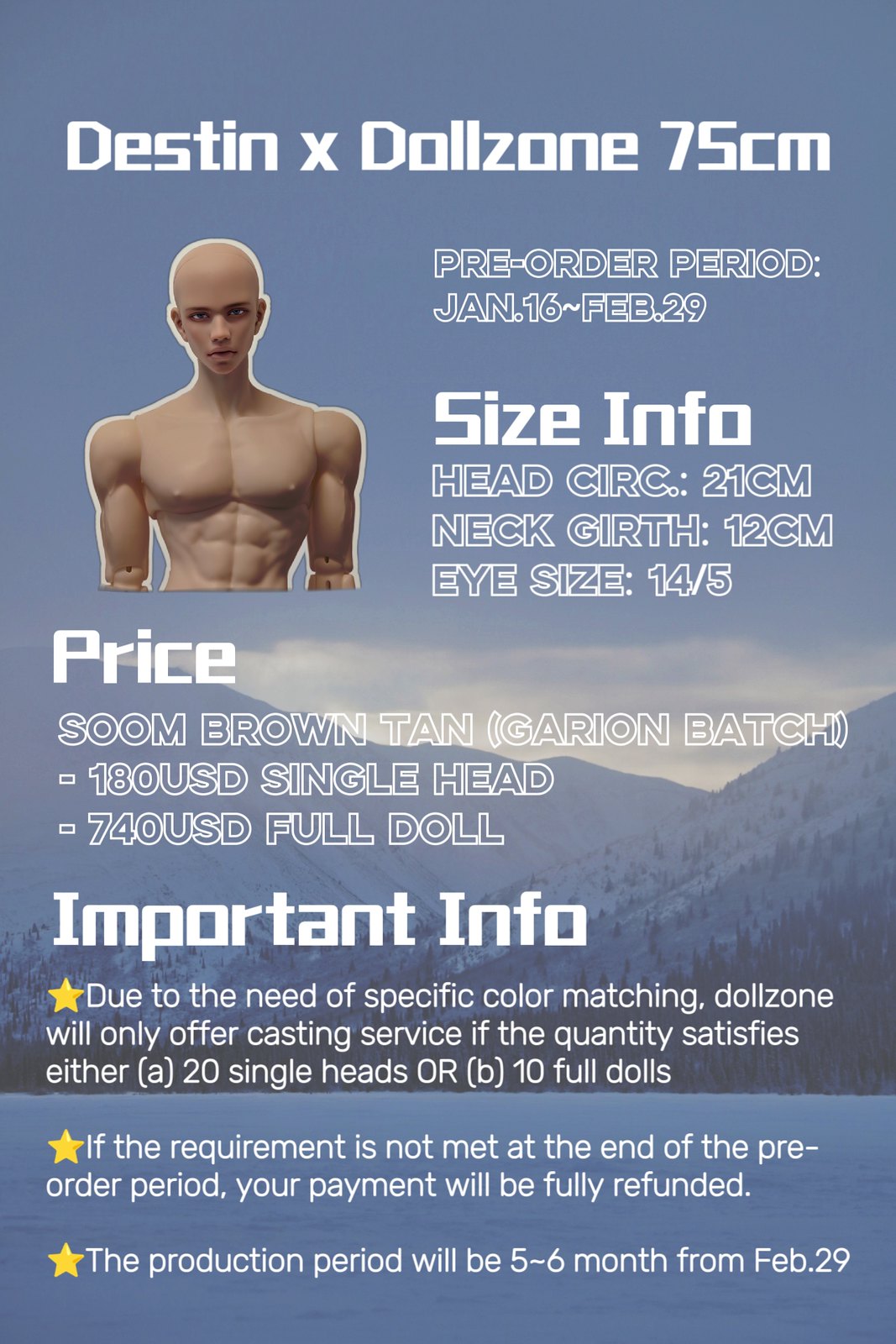The image is an informational brochure for a doll company, titled "Destin X Doll Zone." It announces a pre-order period from January 16th to February 29th for a 75 cm doll. The text details the various size measurements, including a 21 cm head circumference, a 12 cm neck girth, and eye dimensions of 14x5. Pricing is stated as $180 USD for a single head and $740 USD for a full doll, described as being available in a 'brown tan agrarian batch.' The brochure emphasizes that due to the need for specific color matching, Doll Zone will offer casting services if a minimum order of either 20 single heads or 10 full dolls is met. If these requirements are not satisfied by the end of the pre-order period, payments will be fully refunded. The estimated production period is 5-6 months from February 29th.

Visually, the top left of the brochure features an image of the doll, depicted as a muscular, shirtless mannequin with a bodybuilder physique. The text is in white and set against a blue background. Additionally, there is a depiction of a mountain within the background design. The layout of the brochure follows a vertical rectangular shape with the title at the top and the doll image slightly below and to the left. The overall style conveys a polished product advertisement.